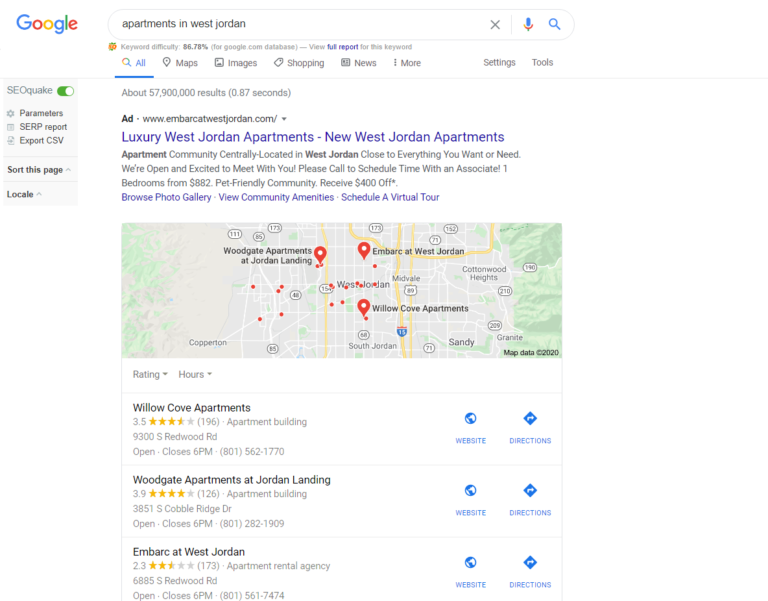This is a detailed screenshot of a Google search page displaying results for "apartments in West Jordan." Dominating the upper left corner is the iconic Google logo, featuring its familiar blue, red, yellow, and green colors. The search bar, centrally aligned and extending toward the right, prominently displays the query "apartments in West Jordan." On the extremity of the search bar, there are two icons—the microphone symbol on the far left side of this area, followed by the magnifying glass icon on the right. 

Directly beneath the search bar, an informational message indicates "Keyboard difficulty 86.78%. For Google.com database, view full report for this keyboard." 

Below this, the search results are listed, with the top entry designated as an advertisement. This first result is for luxury apartments in West Jordan and is from the website www.mbarkatwestjordan.com. The advertisement includes a detailed map pinpointing the location of these apartments and provides ratings for various apartment complexes mentioned within this query.